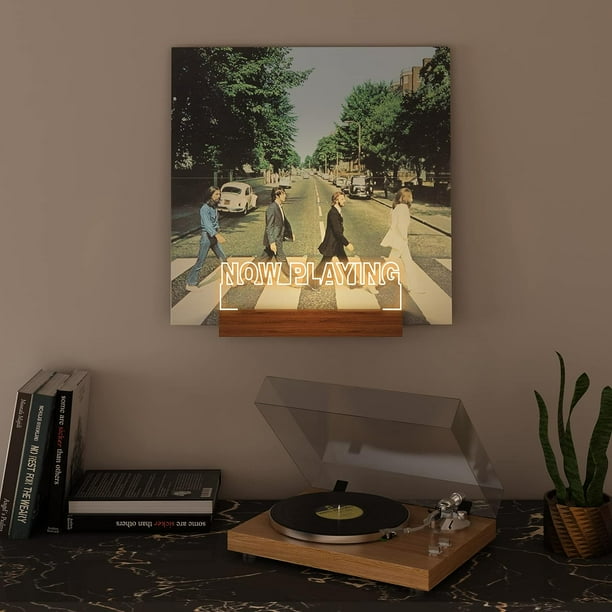The image depicts a well-decorated room featuring a light brown wall as the background. Dominating the wall is a wooden shelf displaying an enlarged Beatles album cover, showcasing the iconic scene of the band members walking single file across a crosswalk. Below the album cover, a small, lit-up sign reads "Now Playing." 

The primary focus is on a presumed granite countertop that spans the width of the scene. On the left side of the countertop, there are three upright books leaning against two books that have fallen over. Moving to the center of the frame, there is a record player with a wooden base and a clear, open top, loaded with a vinyl record. To the right of this turntable sits a plant, sprouting four leaves from the soil. The overall aesthetic combines a retro vibe with modern elements, creating a visually appealing and harmonious setup.